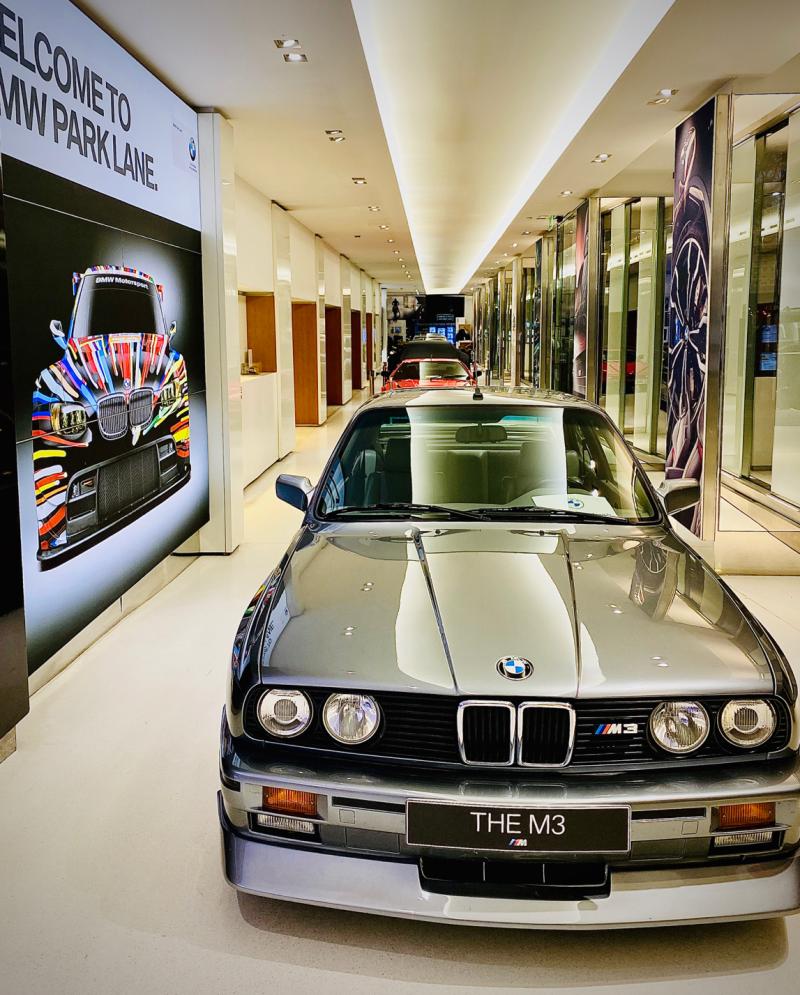The photo captures a pristine BMW showroom with a luxurious ambiance. At the center of the image, a shiny silver BMW M3 is prominently displayed with a reflective hood showcasing the polished lighting above. The car, facing forward, features the distinctive BMW emblem and a front license plate that reads "the M3." An ad to the left welcomes visitors to BMW Park Lane, displaying a vibrant, custom-colored BMW with bright reds, yellows, and blues. The showroom's elegant design includes white flooring, walls, and ceiling, along with detailed pot lights, enhancing the sophisticated atmosphere. Towards the back, the showroom features additional BMWs lined up, including a partially visible red sedan and another dark-colored vehicle. The left side of the showroom is punctuated with wooden cubicles, adding a touch of warmth to the otherwise sleek, white interior. The glass-textured pieces along the right-hand side, possibly showcasing car-related images, contribute to the modern and upscale setting. The overall scene exudes a high-end, meticulously maintained space designed to highlight the featured BMW masterpiece.